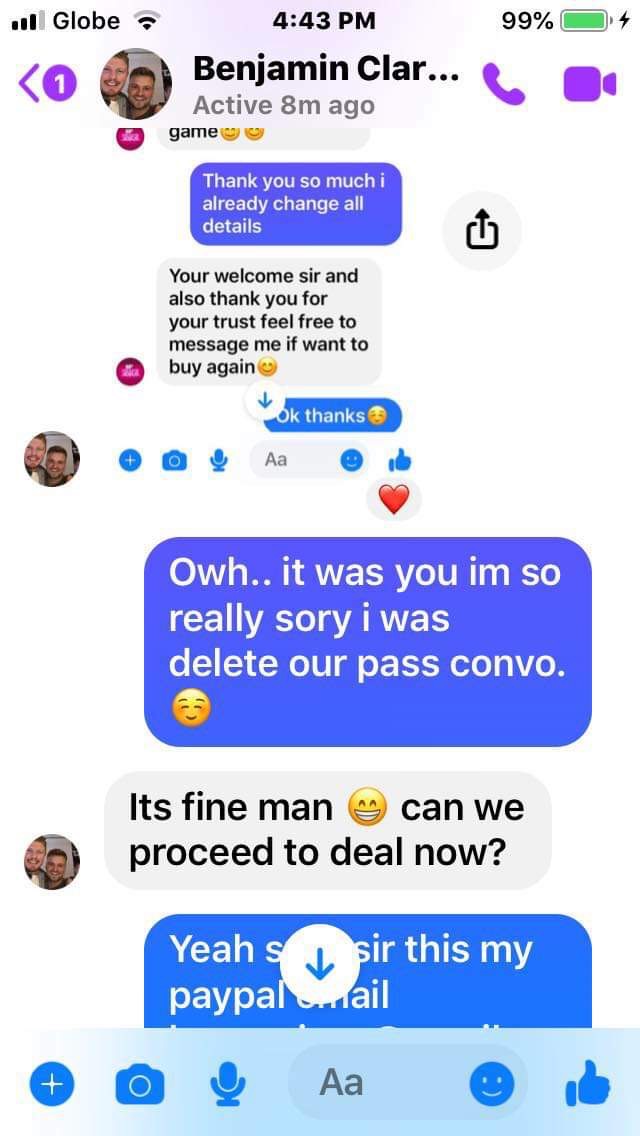This image is a detailed screenshot of a smartphone's messaging app showing a chat conversation with a contact named Benjamin Klar. At the top of the screen, the status bar includes a Wi-Fi indicator, the time "4:43 p.m.", a battery meter at 99%, and the word "Globe" in the center. Immediately beneath the status bar is a header featuring an avatar of two men, the name "Benjamin Klar" with the status "active eight minutes ago", and icons for phone and video calls.

The chat conversation visibly captures a series of back-and-forth messages between the user and Benjamin. The exchange starts with a blue text bubble stating, "Thank you so much. I already changed all details," followed by a gray text bubble replying, "You're welcome, sir. And also thank you for your trust. Feel free to message me if you want to buy again." Another response in gray says, "OK, thanks." Further down, in a blue background, a message reads, "Oh it was you. I'm so really sorry. I was delete our past convo :)". The gray response follows, "It's fine man :), can we proceed to deal now?" The final blue message says, "Yes, [something] sir. This is my PayPal email."

The conversation includes casual gratitude, apologies, and details surrounding a transaction, indicated by the mention of PayPal. There are also several emojis used to convey emotions, including a smiley face and a heart.